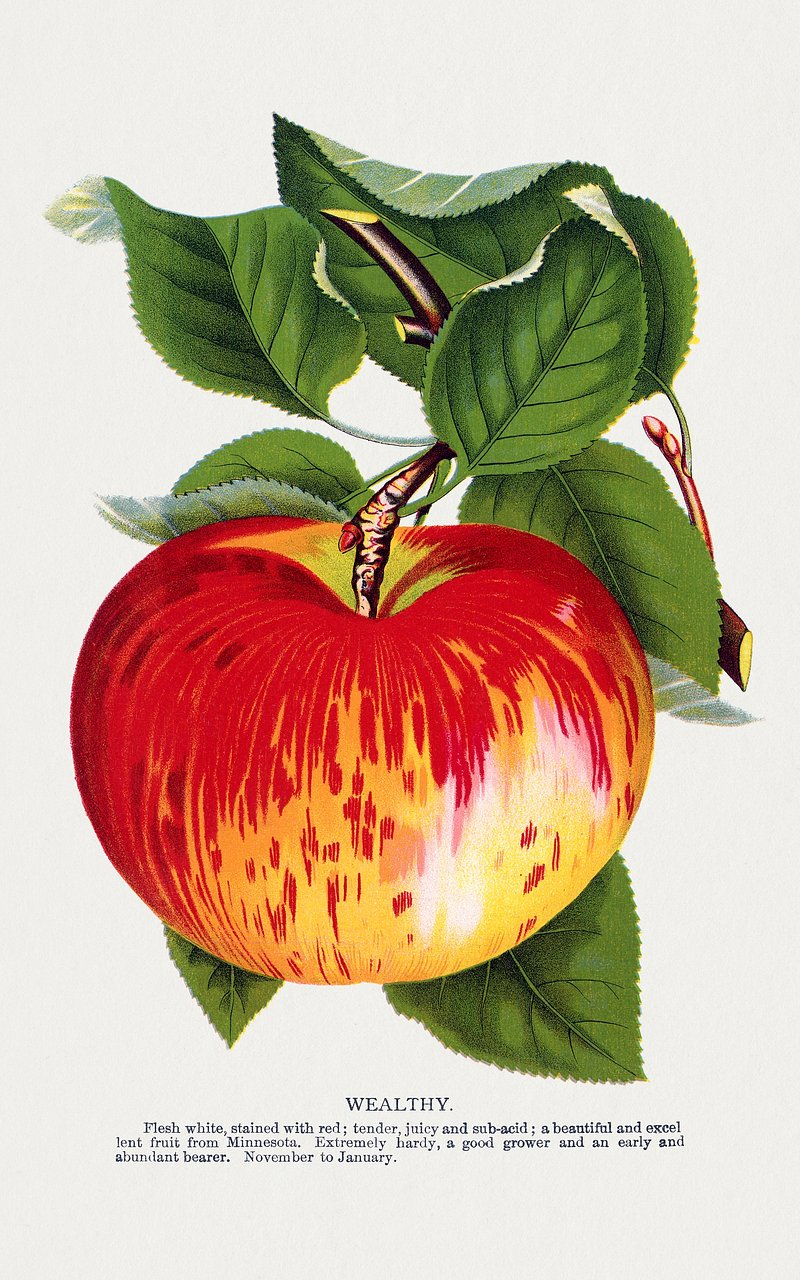The image features a detailed, realistic color illustration of an apple on a white rectangular mat. The apple, which is depicted growing on a stem with green leaves, has a distinctive appearance: it is reddish with a yellow mottling at the bottom and is slightly flatter and donut-shaped compared to typical apples. The illustration has a vintage, etching-like quality and is meticulously detailed, showing not just the apple, but also the stem and the leaves attached to it.

Below the illustration, in bold, black text, it reads "WEALTHY." Beneath this, in smaller type, there is a detailed description of the apple: "Flesh white, stained with red, tender, juicy, and subacid. A beautiful and excellent fruit from Minnesota. Extremely hardy, a good grower, and an early and abundant bearer. November to January." This description highlights the apple's unique qualities and its origin from Minnesota, indicating its resilience and productivity during the colder months.